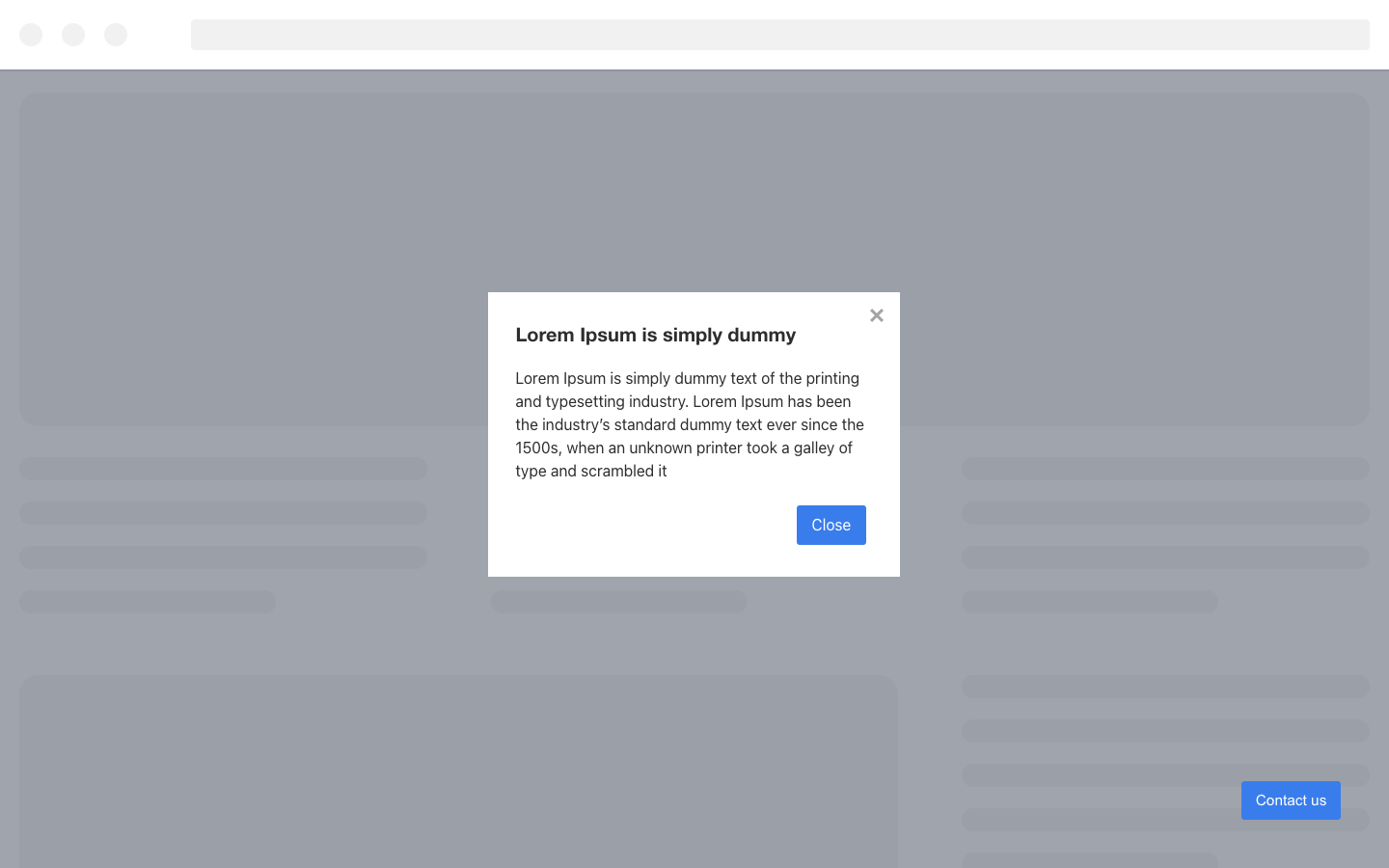A screenshot displays a predominantly grayed-out webpage. At the very top, there is a light gray navigation bar, which is blank except for three small circles aligned to the left. Below this navigation bar, the main section of the page is filled with various placeholder elements. These elements include large gray rectangles representing potential banners or images, and narrower gray rectangles indicating where text might be placed.

Centrally located on the page is a white dialog box with the header "Lorem Ipsum is simply dummy," followed by a paragraph of placeholder text: "Lorem Ipsum is simply dummy text of the printing and typesetting industry. Lorem Ipsum has been the industry's standard dummy text ever since the 1500s when an unknown printer took a galley of type and scrambled it." At the bottom right of this dialog box is a blue button labeled "Close."

In the overall grayed-out page layout, another prominent feature is a blue "Contact Us" button situated at the bottom right corner. The composition of the screenshot suggests it might be a wireframe or mock-up of a webpage, primarily used for design and layout purposes.